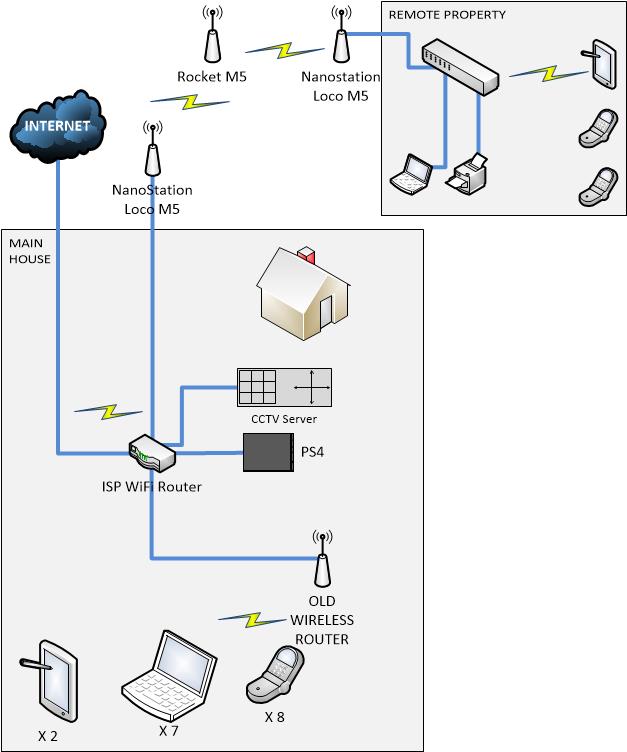The network diagram illustrates the setup for a home network with remote capabilities. In the upper left, a blue cloud labeled "Internet" connects down to the "Main House," depicted with a picture of a house. The connection flows through a NanoStation Loco M5 antenna, into an ISP Wi-Fi router marked by a small lightning bolt. This router links to a CCTV server, a PS4, and an old wireless router. The diagram indicates connectivity for various devices including two tablets, seven laptops/computers, and eight phones.

On the upper right, labeled "Remote Property," another NanoStation Loco M5 antenna connects wirelessly from the "Main House." This connection extends to a remote box labeled "Remote Property," which links to a printer and another computer, and supports one tablet and two phones. The visual representation is akin to those found in instruction manuals for setting up a router, with clear labels and connections illustrating the flow and structure of the network.